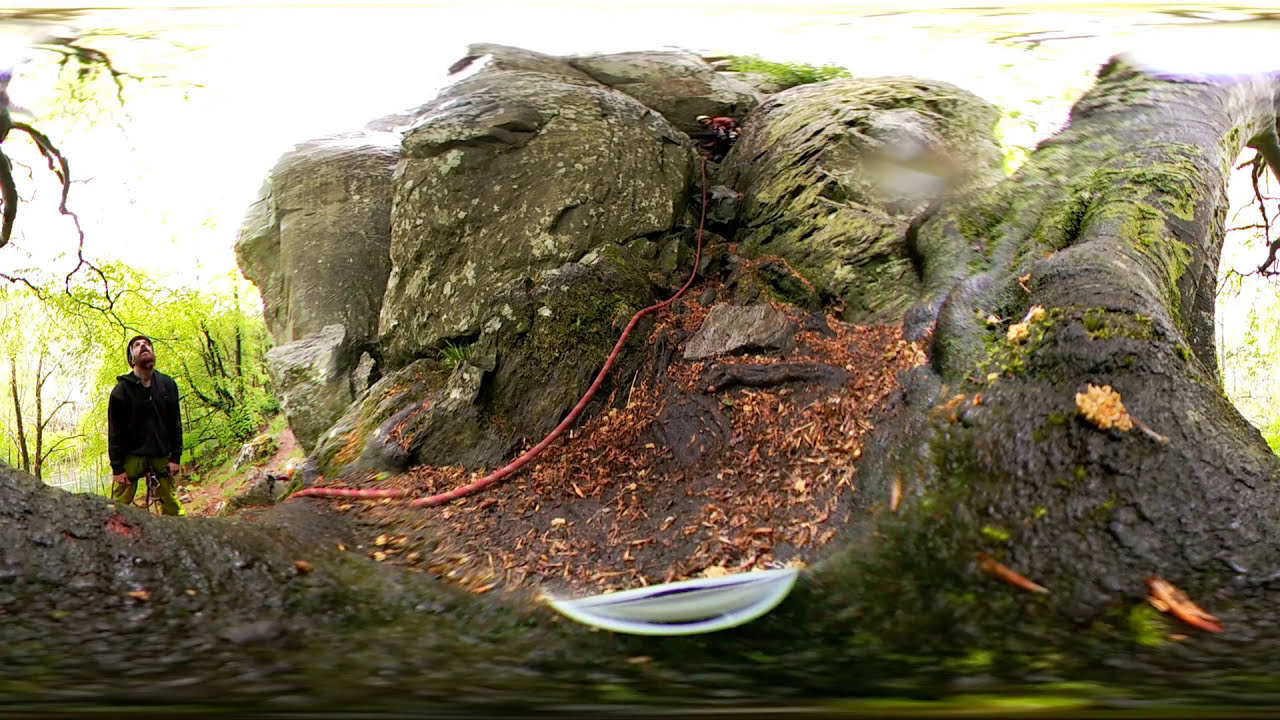The photograph showcases a rugged outdoor scene dominated by a substantial rock formation situated next to a slightly angled tree on the right side, which appears to be old and covered in green growth. At the summit of the rocky structure, a climber wearing a red shirt and white helmet is seen near the top of a red rope with lighter stripes running through it. This rope stretches all the way to the ground where another man, identifiable by his black jacket, beanie hat, and beard, stands on a dirt path. This man, who is also equipped with a climbing harness, gazes upward attentively towards the climber. The backdrop features lightly leafed green trees interspersed with sunlight, indicative of early spring, and the forest floor is scattered with remnants of leaves from the previous winter. The image, likely taken with a 360-degree camera, captures the depth and complexity of the scene, emphasizing the connection between the towering natural rock formations and the active climbers navigating them.